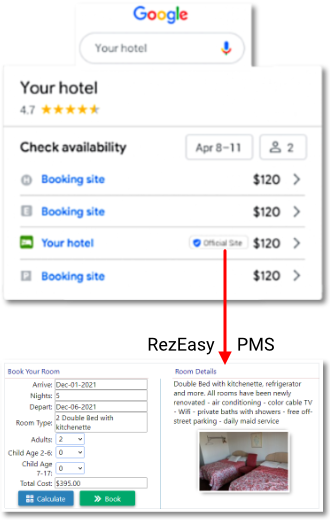This vertically oriented image appears to be a screenshot from a smartphone, taken against a plain white background, likely the user's computer screen. At the very top, a rectangular box displays the Google logo in its traditional multicolored letters (blue, red, yellow, blue, green, red). 

Directly below this, a rounded rectangular search bar reads "Your Hotel" in gray text, accompanied by a microphone icon on the right. Beneath the search bar, a larger rectangular section features "Your Hotel" in black text, followed by a 4.7 rating illustrated with yellow stars. This section is separated by a thin gray line from the subsequent text in bold black: "Check Availability." 

Adjacent to the "Check Availability" text, a small box displays the dates "April 8th through 11th," and another box shows an icon representing a person alongside the number 2, indicating the number of guests.

Below the availability section, four icons in blue each read "Booking Site, Booking Site Your Hotel, and Booking Site." Each listing is accompanied by the price "$120." The “Your Hotel” listing is distinguished by the label "official site" next to a red downward arrow labeled "Res Easy PMS." Room details are provided in blue text, followed by additional information in black and an image of the room. 

On the left-hand side, a "Book Your Room" section includes fields for inputting booking information and calculating costs, concluded with a green "book" button.